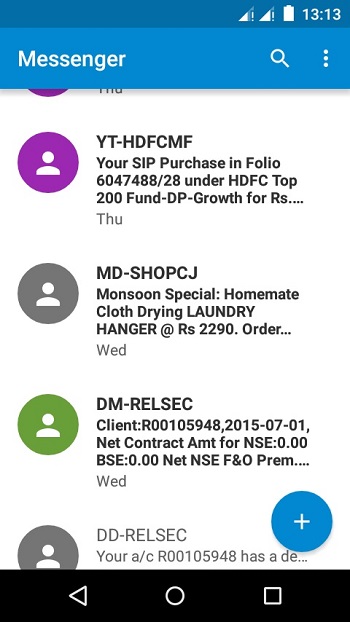A cell phone screenshot of a messaging app is the focus of the image. At the top, within a blue rectangular banner, the word "Messenger" is displayed in white text. To the right of this banner, there is a magnifying glass icon representing the search function, followed by three vertical white dots indicating additional options.

Moving down, the screen displays a series of contact icons, each represented by circles with simplified human figures (a round head and a semicircular torso). The very top contact icon is purple but is partially obscured by the "Messenger" banner. 

The next visible contact icon is also purple and prominently displays the text "YT-HDFCMF" in capital letters. Below this, it reads: "Your SIP purchase in folio 6047488-28 under HDFC Top 200 Fund-DP-Growth for RS..." in smaller font, with "THU" in gray print indicating the time or day of the message.

Following this, a sequence of contact icons appears: a gray circle with a human silhouette, a green circle, and another gray circle, before the visible part of the screen ends. At the very bottom, a black bar features navigation icons—a triangle, a square, and a circle—indicating the typical Android phone navigation buttons.